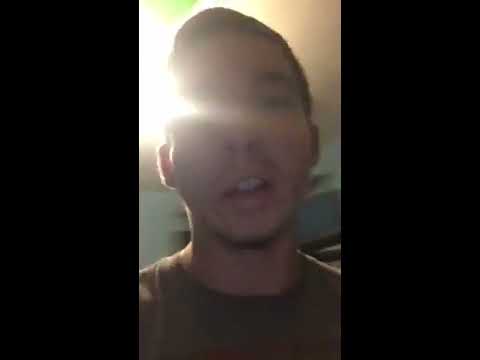The image appears to be a selfie taken indoors, possibly during a FaceTime call, showing a young white male with dark, short hair styled in a buzz cut. His face is very close to the camera, and there's a bright light fixture behind his head, casting a light that partially obscures his right eye. He is wearing a dark t-shirt, which seems to be either dark brown, dark gray, or military green. The background reveals a white ceiling and bluish-green walls, with some large, indistinct dark objects. The man appears to be in the middle of speaking, given his slightly open mouth, and there is a shadow or possibly facial hair under his chin. The overall setting suggests a casual indoor environment, likely his home. The presence of black borders on the sides of the image imply it could be a screenshot from a FaceTime call.